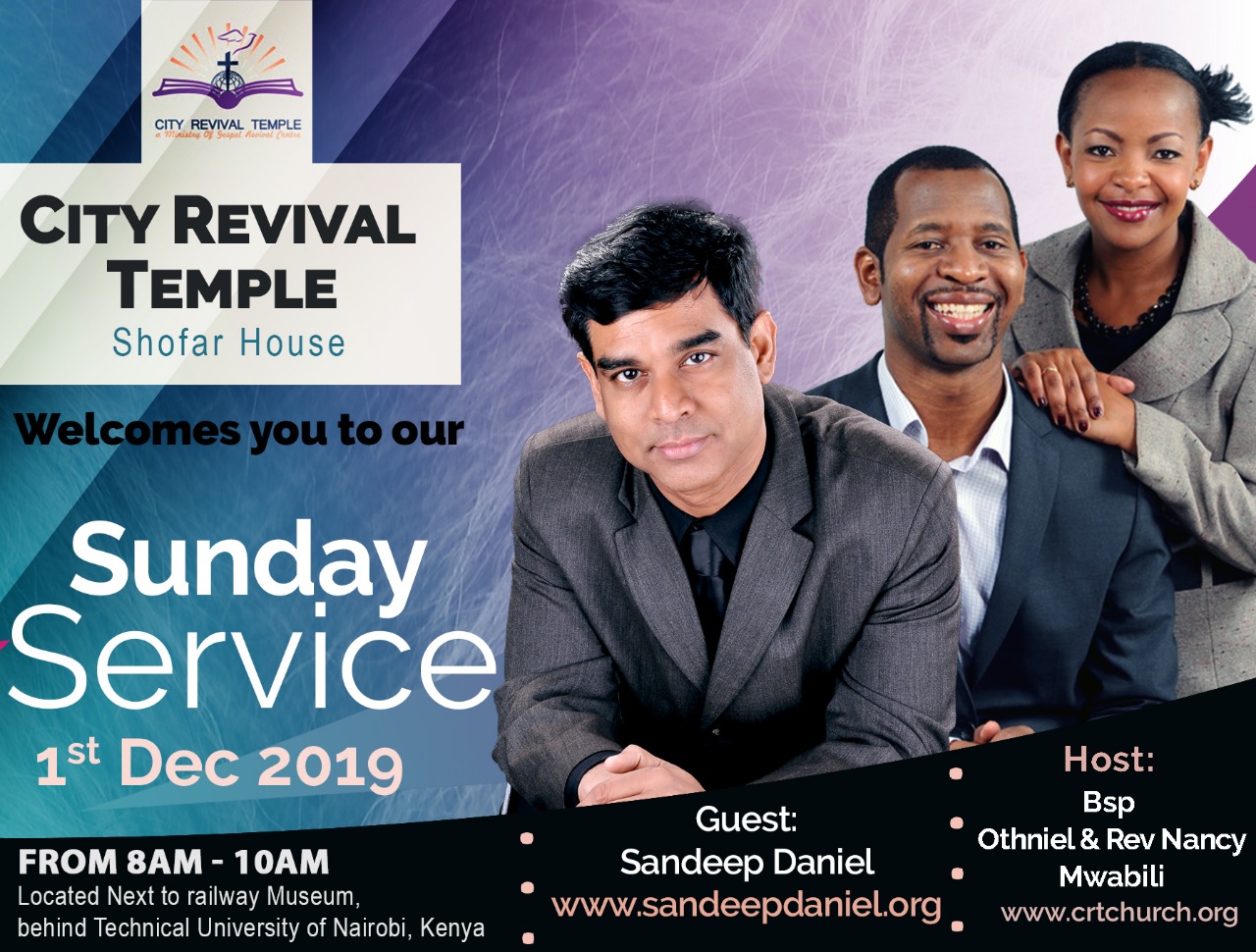The poster for City Revival Temple's Sunday service on December 1st, 2019, features a detailed and inviting design. In the top left corner, there is a logo of the church, depicting a cross over an open purple book with yellow sun rays, accompanied by the text "City Revival Temple, Shofar House." The central part of the poster warmly invites everyone to their Sunday service. 

Dominating the right side of the image are three individuals. Centered is a Middle Eastern man with black hair, dressed in a gray suit, black shirt, and black tie, gazing straight ahead. To the left and slightly behind him is an African American man wearing a blue blazer and light blue button-down shirt, smiling broadly. Beside them, a woman with short black hair, dressed in a brown suit jacket and a black necklace, also smiles warmly, her hands gently resting on the shoulder of the man in the blue suit. 

The bottom section of the poster is set on a black background and provides further details about the event, including the service time from 8 a.m. to 10 a.m., guest speaker Sandeep Daniel with a link to his website (www.sandeepdaniel.org), and the hosts, BSP Othniel and Reverend Nancy Mwabili, with a mention of the church's website (www.crtchurch.org). The overall design transitions from black text to white and a hint of pink, creating an eye-catching and informative layout.